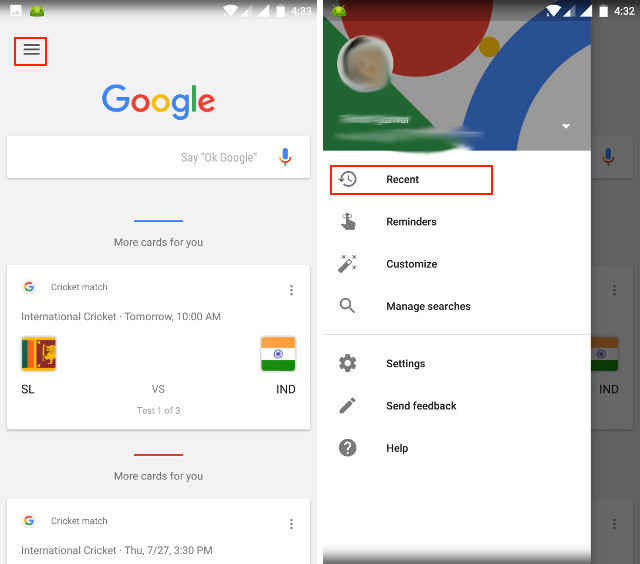The image is composed of two adjacent screenshots from a mobile phone displaying different Google-related interfaces. The left screenshot features a Google search page. At the top of this page is the Google logo with a search bar below it. Inside the search bar, the text "Say 'OK Google'" is visible, accompanied by a microphone icon to its right. Beneath the search bar, a grey separator reads "More cards for you," followed by a white notification card. This card has a Google icon on the top left and, next to it, the text "Cricket match." Below this, it reads "International cricket tomorrow at 10 a.m.," indicating a match between Sri Lanka (SL) and India (IND). Another card below it mentions a cricket match scheduled for Thursday from 7:27 to 3:30 p.m.

The right screenshot displays a Google+ profile interface in what appears to be the poll window. The avatar at the top of this window is pixelated, making it indistinguishable. Below the avatar, there is a vertical list of options. The first option, "Recent," is highlighted with a red box. The subsequent options, which are not highlighted, include "Reminders," "Customize," "Manage searches," "Settings," "Send feedback," and "Help."

This detailed juxtaposition of the Google search and Google+ profile page captures the interface and functionalities of the mobile Google ecosystem.